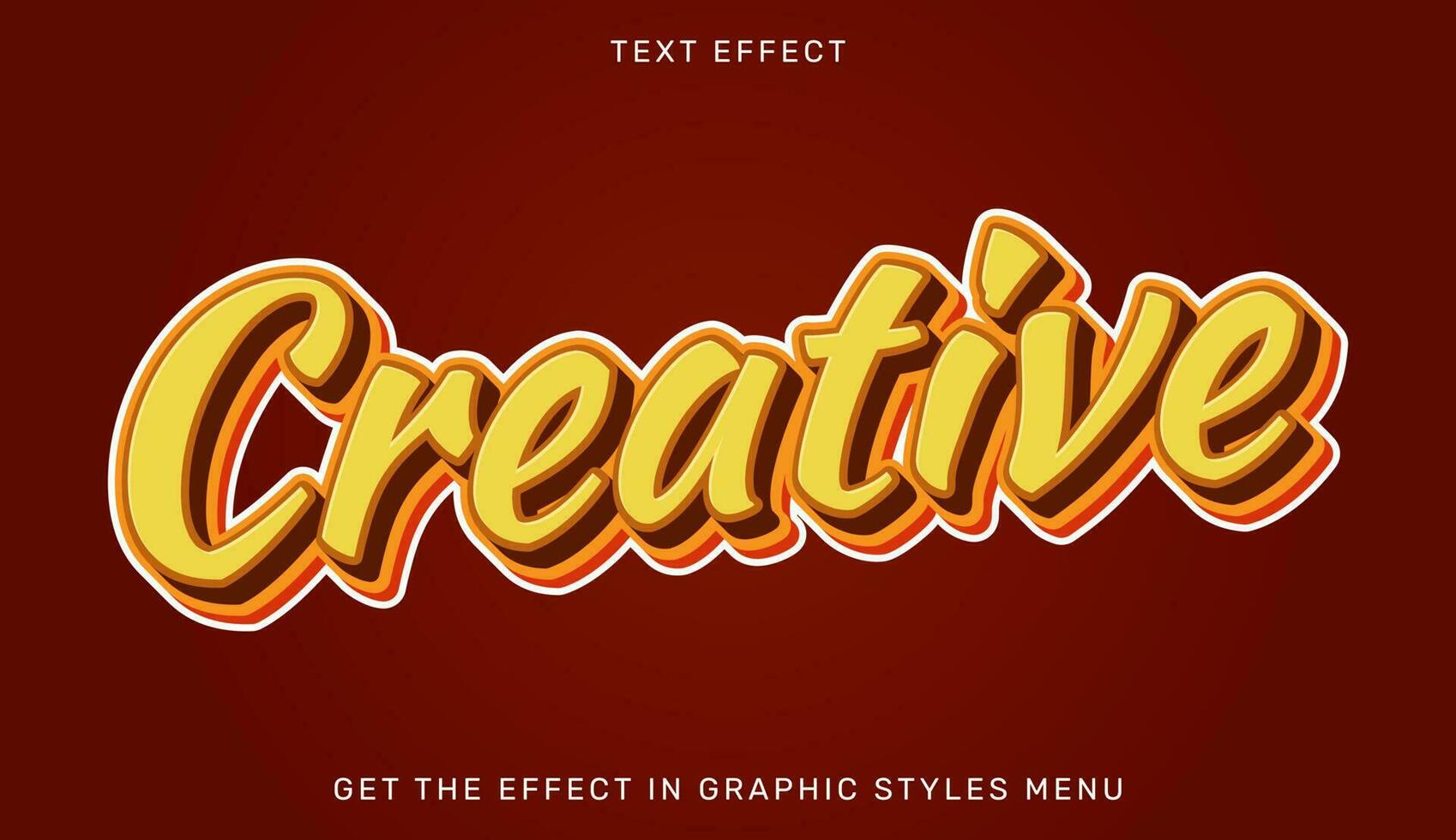The image features a simple yet striking graphic design set against a reddish-brown, almost maroon background. The center of the image is slightly lighter, creating a subtle spotlight effect. At the top in very small, all-caps white font, it reads "TEXT EFFECT," while at the bottom, also in small, all-caps white font, it reads "GET THE EFFECT IN GRAPHIC STYLES MENU." Dominating the center is the bold word "CREATIVE" in large, 3D-styled letters. The word "CREATIVE" features layered colors—yellow on top, followed by layers of light brown, orange, darker orange, with a prominent white outline that enhances its 3D effect. The overall dimensions resemble that of a high-definition television, suggesting it could be a screenshot from a computer screen, particularly from a graphic design software's menu showcasing text effects.